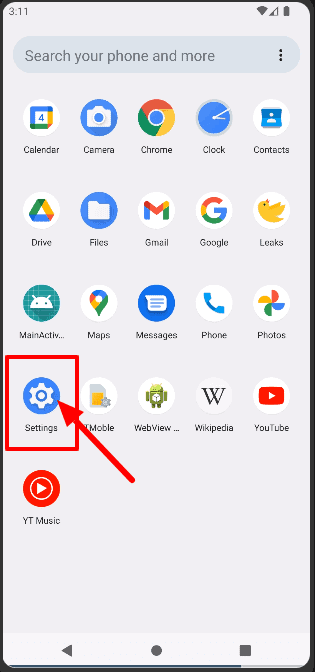The image depicts a smartphone home screen showcasing a variety of app icons arranged in a specific order. The apps are organized alphabetically from top to bottom and right to left. At the top of the screen, the visible apps include Calendar, Camera, Chrome, Clock, and Contacts. Continuing downward, the next row features Drive, Files, Gmail, Google, and an app named Leaks, which is illustrated with a yellow bird resembling a deceased Twitter bird, complete with 'X' eyes.

Further down, the apps include Main Active (with ellipses indicating the name might be truncated), Maps, Google Maps, Messages, Phone, Photos, Settings, T-Mobile, Web View, Wikipedia, YouTube, and YouTube Music. Notably, the Settings app has a box drawn around it and a red arrow pointing to it, suggesting it has some particular importance or needs attention. The detailed layout and annotations on the screen indicate a highly organized and possibly curated selection of apps for the user’s convenience.